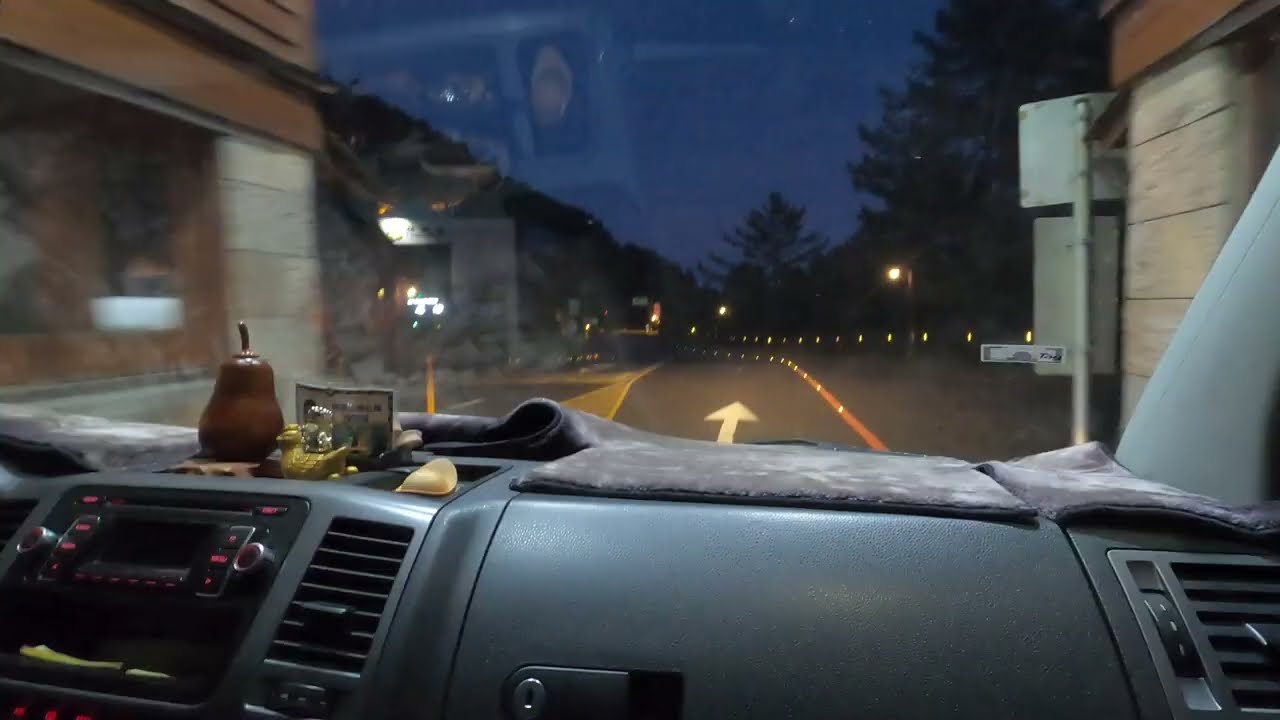The photograph, taken from the perspective of a passenger inside a car at night, captures a one-way roadway ahead, with an upward-pointing arrow clearly visible. The shot provides a partial view of the car's interior, showing the dashboard to the left, which features a radio and some gray lining, possibly resembling a carpet sample. Notably, a decorative pear rests atop the dashboard. The sky outside is dark but not completely black, illuminated by streetlights that also cast light on the scene, allowing for trees to contrast against the sky. The road, flanked by indistinct buildings, is well-lit and occupies the center of the image. The car's interior showcases a mix of blue, aqua, and gray tones, while the entire photo features a detailed array of colors, including brown, white, gray, red, black, tan, yellow, and dark blue. The absence of text keeps the focus on the visual details within and outside the vehicle.